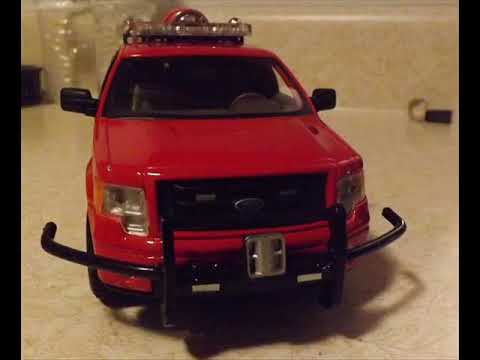The image depicts a detailed scene with a vibrant red toy truck, resembling an emergency vehicle, prominently displayed on a beige countertop or vanity top. The truck features a black bumper bar attached to the front with a silver square plate and has black side mirrors. A blue Ford emblem adorns the center of its black grille, and clear headlight covers flank the emblem. Atop the truck, a silver tray holds a semi-circular object with a red rim, while silvery white bar lights are also visible. The interior of the truck’s cab, though somewhat shadowed, reveals the steering wheel and the passenger side backrest. 

The background showcases a predominantly yellow color with a black backsplash. In the back left corner, there are two plastic water bottles and a black object partially off-screen. To the right, the floor is adorned with a black box and what looks like an ice cube. Additionally, in the top left corner, a black chair stand is visible near the wall. The entire image is framed by a narrow black border on the left and right sides.